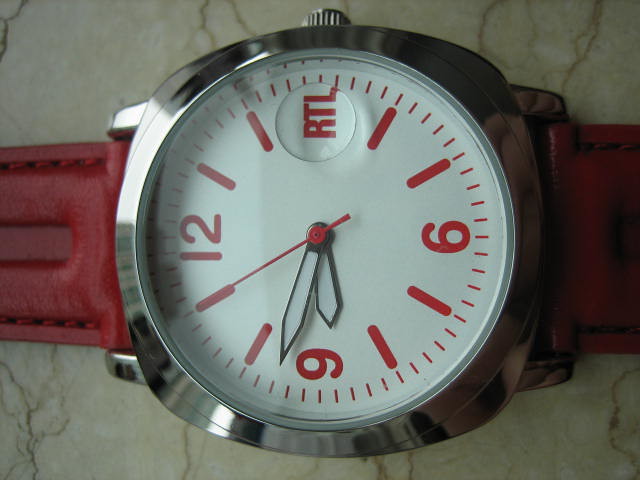In this detailed close-up photograph of a wristwatch, the watch is oriented with its top facing left and its bottom right, laying on what appears to be a light gray marble countertop with light brown veining. The timepiece features a striking red leather wristband and a stainless steel bezel encircling its white dial. Prominently displayed on the face, the numerals 12, 6, and 9 are depicted in red, while other hour markers are indicated by simple red lines accompanied by smaller red lines for the minutes. Notably, the area where the numeral 3 would be is marked with the text "RTL." The watch hands are white, with the second hand in red, currently showing the time at 8:53 and 55 seconds. The image appears slightly rotated to the left, adding to the unique angle of the shot.